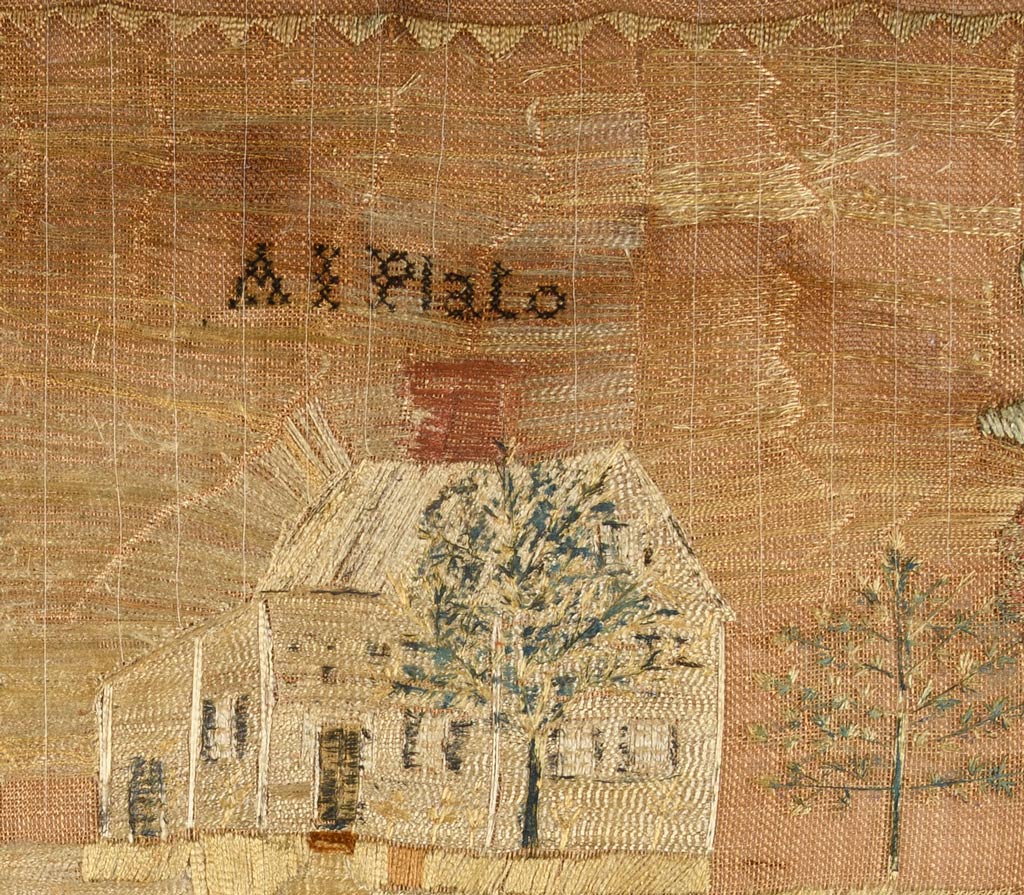The image depicts an aged, hand-sewn textile piece that features intricate embroidery on a rustic beige and brown burlap-like fabric. Central to the design is a one-story cream-colored prairie house with a distinct roof, two doors, and three windows—notably, one with black shutters. The embroidery threads, now worn and faded, include hues of darker copper, light white, yellow, and teal. In front of the house, a sparsely defined tree with a dark brown trunk and branches adorned with blue and pale yellow leaves adds character, while another, more discernible tree with a slender black trunk and branches sporting faded green and yellow leaves stands to the house's right. Additionally, black stitched text, which appears to read "A L P L A T O," is visible but heavily worn, adding to the piece's antique and rustic charm.